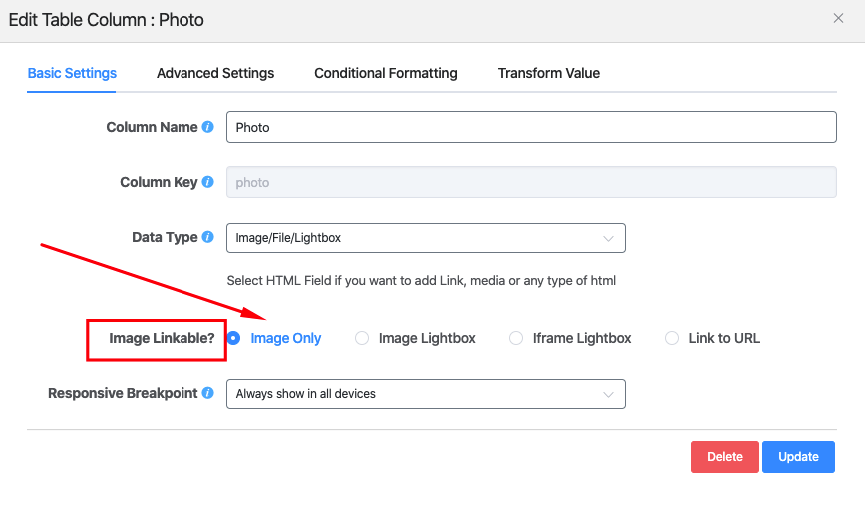This screenshot captures the interface of an edit table column settings dialog. At the top, a gray header displays "Edit Table Column" in black text, followed by "Photo" to the right, indicating the column being edited. An 'X' icon is located at the far right for exiting the dialog.

Directly below the header, a navigation bar categorizes the features into tabs: Basic Settings (highlighted), Advanced Settings, Conditional Formatting, and Transform Value. The content shown pertains to the Basic Settings tab.

Under Basic Settings, the "Column Name" field is presented first, accompanied by an information icon (blue eye icon) to the right. This field contains the text "Photo" within an editable text box. Following that is the "Column Key," which also features an information icon and a grayed-out text box with "photo" filled in, indicating it is not editable.

Next, the "Data Type" field displays "Image File Lightbox" as its value. Centered below in gray text, a message explains: "Select HTML field if you want to add link media or any type of HTML."

At the bottom left is an option labeled "Image Linkable" with a red box highlighting the area and a red arrow pointing to a "Image Only" selection, which is highlighted in blue. This indicates that only the image is linkable in this configuration.

Finally, at the bottom right of the screenshot are two buttons: a red "Delete" button and a blue "Update" button, allowing the user to either remove or save the changes made to the column settings.